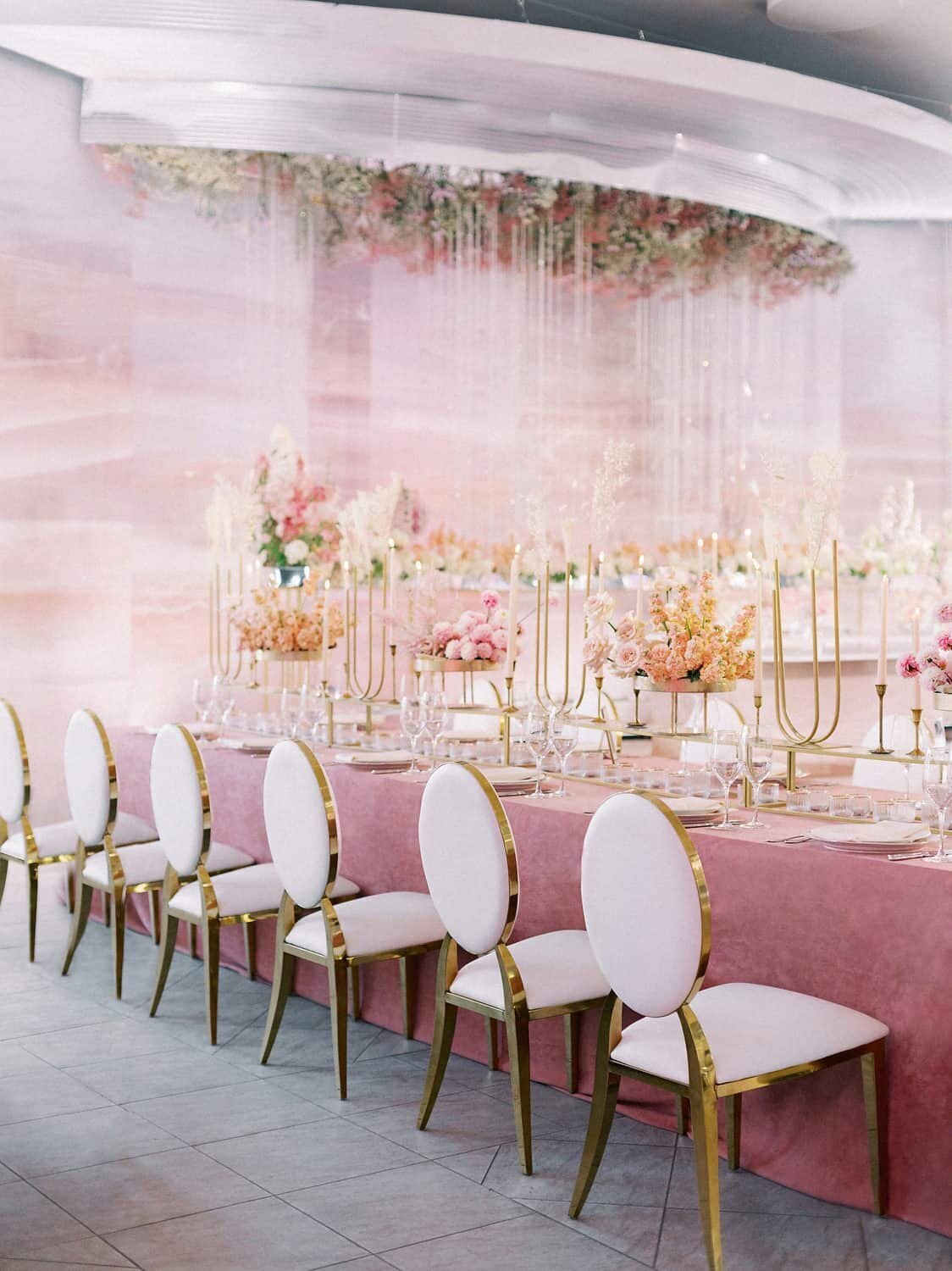This photograph captures the opulence of a formal event, likely a wedding or bridal shower, held in an elegantly decorated banquet room. The prominent feature is a long banquet table adorned with a floor-length pink tablecloth and set with six elegant white and gold chairs, each with white oval backs bordered in gold and matching white seat cushions on gold legs. The table is meticulously set with formal serviceware, including multiple plates, silverware, and two glasses at each setting, likely for wine and water. The centerpiece features a table runner embellished with ornate floral arrangements composed of pink, orange, and yellow blooms, likely including mums, roses, and carnations, interspersed with tall candle holders bearing long candles. Adding to the grandeur, a decorative chandelier with hanging crystals and flowers is suspended above the table, casting a delicate and whimsical light over the entire scene. The background, though blurred, hints at additional tables and floral arrangements, as well as perhaps some traction installations that allow plants to hang from the ceiling or walls, enhancing the dreamy atmosphere of the room.